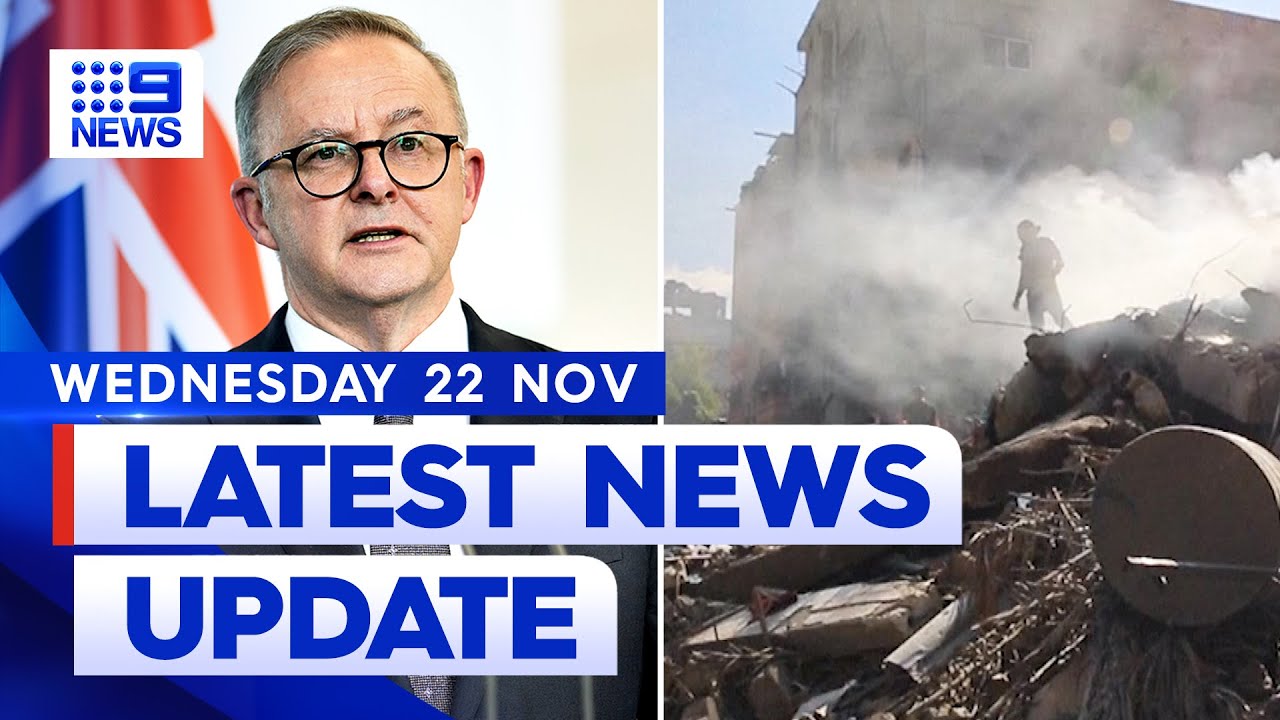In the screenshot, we are viewing what appears to be a news broadcast, likely sourced from either a website or a video. In the top left corner, the logo "News 9" is prominently displayed in blue. The screen is split into two segments.

On the left-hand side, we see an older man, estimated to be in his late 50s or early 60s. Behind him, there appears to be a flag, possibly a British flag, hinting at his potential association with the UK government. Below him, a banner reads "Wednesday, 22nd November, Latest News Update." The phrase "Latest News Update" is written in blue lettering against a white background, while "Wednesday, 22nd November" is displayed in white lettering on a blue background.

The right-hand side of the screen depicts a chaotic scene, likely the aftermath of a disaster or explosion. A man stands amidst significant destruction, surrounded by heavy smoke and debris. The ground around him is littered with remnants, suggesting a recent catastrophic event.

Overall, this screenshot from News 9's broadcast on Wednesday, 22nd November, features an image of an elderly gentleman, potentially linked to the British government, juxtaposed against the harrowing scene of a recent disaster characterized by an explosion and heavy smoke.